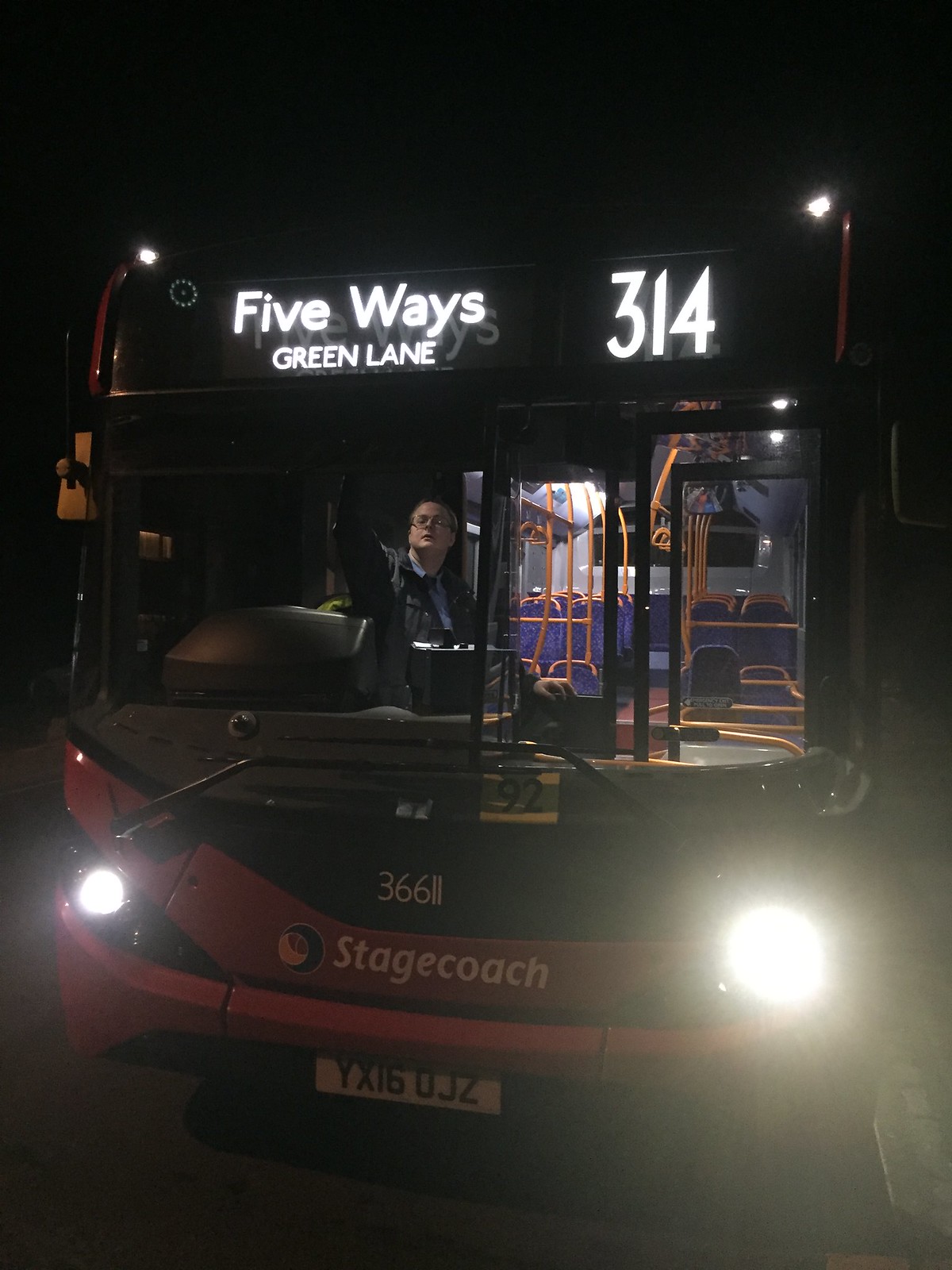In the image, a Stagecoach bus is photographed head-on against the backdrop of a dark night. The bus, with its distinct red body and white lettering, prominently displays the "Stagecoach" name and a circular logo. The headlights are on, casting light on the dark scenery. A detail that stands out is the license plate, YX160JZ, positioned below the front lights. Above, a destination sign reads "Five Ways, Green Lane, 314" in white text against a black background.

Inside the bus, the lighting contrasts with the dark exterior, revealing blue seats and yellow holding bars near the back. The bus driver, a gentleman wearing glasses, is visible through the front window, making a gesture as he looks towards the photographer. Though the bus appears operational with lights on, the driver is not currently driving.